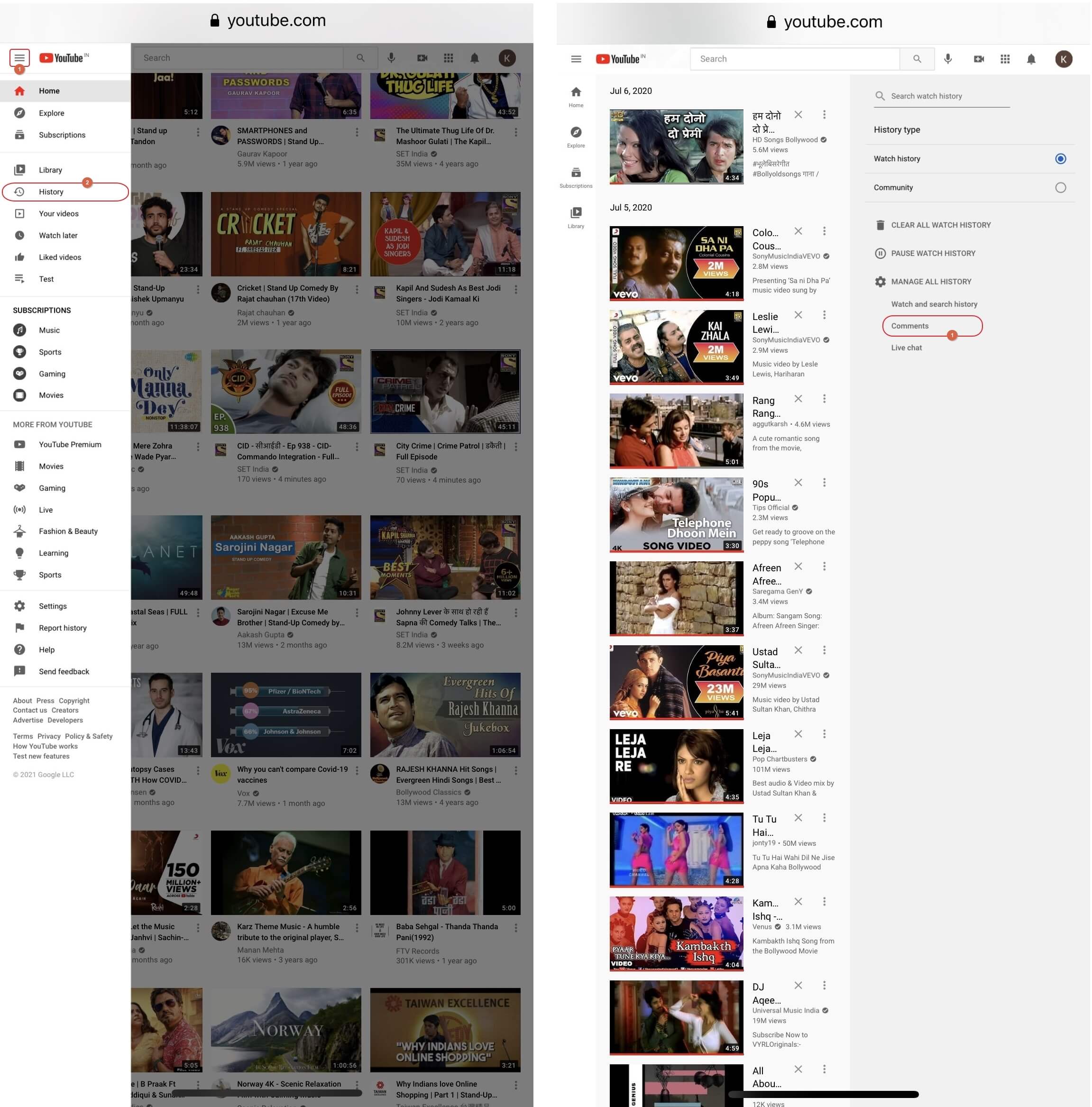The image consists of two different YouTube pages displayed side by side, suggesting it might be from a mobile device due to its tall and narrow shape. However, the absence of typical mobile interface symbols like Wi-Fi or signal bars makes this uncertain.

On the left page, set against a white background, the YouTube logo is prominently displayed alongside a locked padlock icon. Below the logo is a vertical menu listing several options such as Home, Explore, Subscriptions, Library, and History – with History highlighted in red. Additional menu options include Your Videos, Watch Later, Liked Videos, and a category labeled Test. Further down, there are sections titled Subscriptions and More from YouTube, followed by links to Settings, Report History, Help, and Send Feedback. To the right of this menu, the screen is dimmed, showing various video thumbnails that don't seem to share a common theme.

The right page also begins with the YouTube logo and a locked padlock icon at the top. Below, there are similar navigation options: Home, Explore, Subscriptions, and Library. Unlike the left, this page displays a single column of video thumbnails, predominantly featuring Indian content. Some video titles explicitly reference Indian culture, like "Universal Music India" and "Song from the Bollywood Movie," indicating the search results focus on Indian videos. On the far right, there is a menu with options for managing watch history, including Search Watch History, History Type, Watch History Community, Share All Watch History, Pause Watch History, and Manage All History.